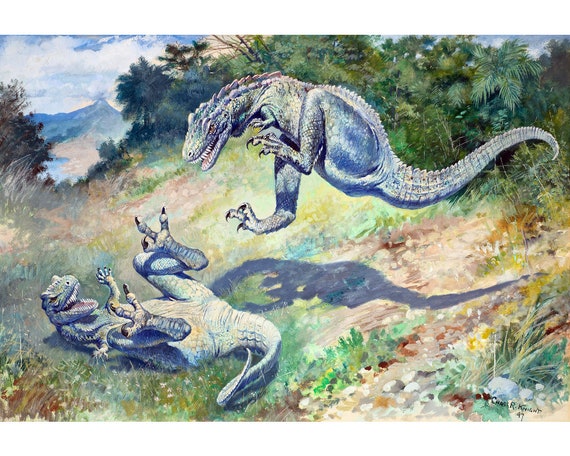This horizontally oriented, cartoon-like image or drawing appears hand-drawn or digitally created. It depicts a dynamic prehistoric scene featuring two T-Rexes either fighting or playfully interacting on a hill covered with green grass, brown dirt, bushes, and plants. The terrain gives way to a background featuring a towering mountain on the left, possibly a volcano spewing steam and red lava. The well-lit scene boasts a blue sky filled with fluffy white clouds.

In the center, the two T-Rexes command attention with their distinctive details. The one on the ground, lying on its back with mouth agape, displays sharp teeth, small hands pointed skyward, and legs raised with its tail coiled. The other T-Rex is mid-air, seemingly about to pounce, with its legs extended, small arms tucked close, and mouth open to reveal its own set of white teeth. Both dinosaurs are green with red tongues and white teeth, though one caption mentions them as bluish gray. Surrounding the central figures, a dense array of green foliage and shrubs adds to the jungle-like setting, emphasizing the Jurassic theme.